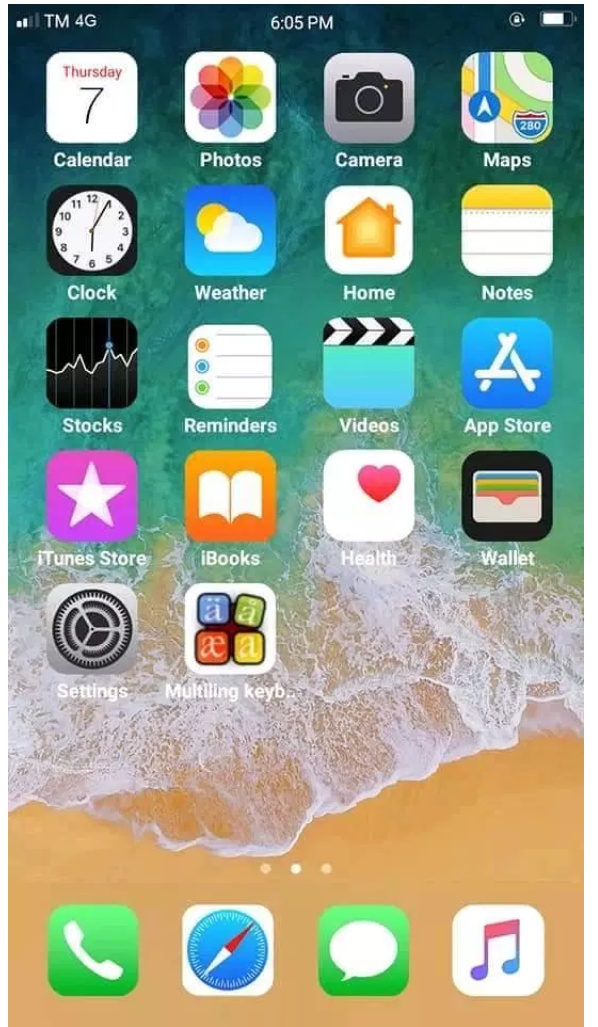This image is a screenshot of a smartphone's home screen, set against a serene beach-themed wallpaper. The wallpaper features a gradient beginning with a sandy shore at the bottom, where foamy, white waves gently caress the sand. As the view extends upward, the tranquil water transitions into a calming, teal-blue sea, evoking a sense of peace and the allure of a perfect beach getaway.

The home screen is organized into five rows of app icons, though the last row only contains two icons while the others each have four. 

At the very top, the status bar indicates it's Thursday the 7th, followed by the first row of apps:
1. **Calendar** - Displaying today's date.
2. **Photos** - Represented by a colorful flower icon.
3. **Camera** - Denoted by a camera icon.
4. **Maps** - Indicated by a map icon.

The second row includes:
1. **Clock** - Featuring a clock face.
2. **Weather** - Depicted by an icon of clouds and a sun.
3. **Home** - Represented by an orange house.
4. **Notes** - Symbolized by a notebook page.

The third row presents:
1. **Stocks** - An app likely dedicated to financial updates.
2. **Reminders** - For managing tasks.
3. **Videos** - Represented by a play button.
4. **App Store** - The platform for downloading apps.

The fourth row displays:
1. **iTunes** - For music and media.
2. **iBooks** - For reading and purchasing books.
3. **Health** - Represented by a heart.
4. **Wallet** - For managing digital payments and cards.

Finally, the fifth row consists of:
1. **Settings** - The app for configuring device settings.
2. **Multilingual Keyboard** - Indicating a tool for multiple language inputs.

Overall, this detailed arrangement of apps against an inviting beach backdrop combines functionality with a visually pleasing aesthetic.